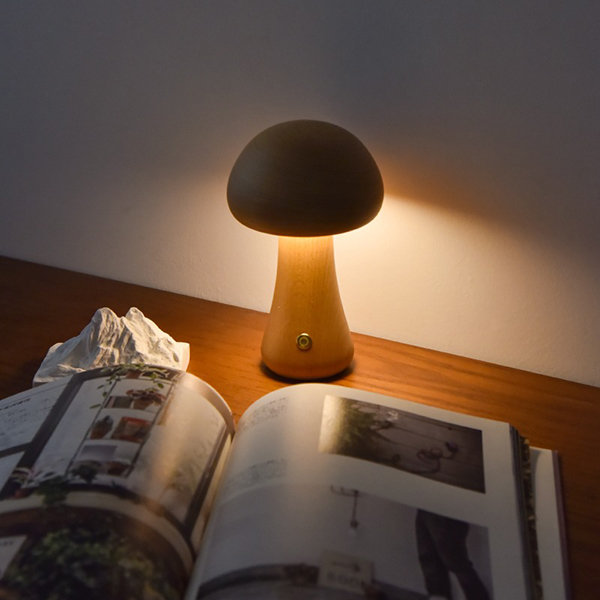The image depicts an intricately detailed scene set against a white wall, featuring a wooden table bathed in dim light. At the center of the table sits an open book, its pages obscured by shadows, though faint glimpses suggest photos of plants and a person's legs clad in pants. To the book's left lies a crumpled white napkin, adding an element of casual clutter. Illuminating the book is a unique desk lamp resembling a wooden mushroom, with a soft light emanating from beneath its cap. The lamp's base features a small, goldish button switch, contributing to the overall subdued and cozy ambiance of the scene.